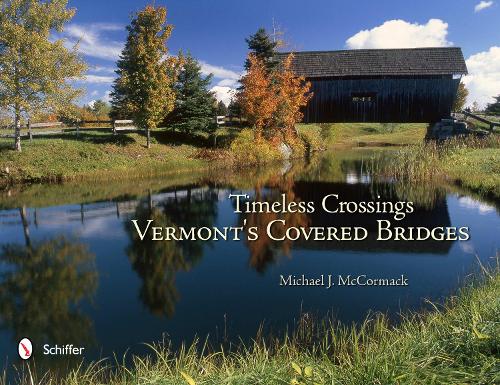The image likely depicts a postcard featuring a picturesque, country setting. Central to the scene is a large, covered bridge with wood siding and black shingles, arching over a serene creek that runs diagonally from the bottom left to the upper right of the image. The water is calm, reflecting the tranquility of the surroundings. In the foreground, there is a stretch of grass, and further in the distance, various trees, including pines and a birch, can be seen alongside a tree with orange foliage, indicating the onset of fall. There's also a small hillside with more trees and a fence stretching across the background.

The bridge itself, distinguished by a small rectangular window and a clear path running through it, adds to the rustic charm of the scene. Above the bridge, the sky is a soft blue with scattered clouds. Across the middle of the image, there is white text reading "Timeless Crossings," followed by "Vermont's Covered Bridges," and the name "Michael J. McCormick." The bottom left corner of the image features a symbol and the word "Schiffer" in white, suggesting that this might be a postcard or informational card celebrating covered bridges in Vermont.